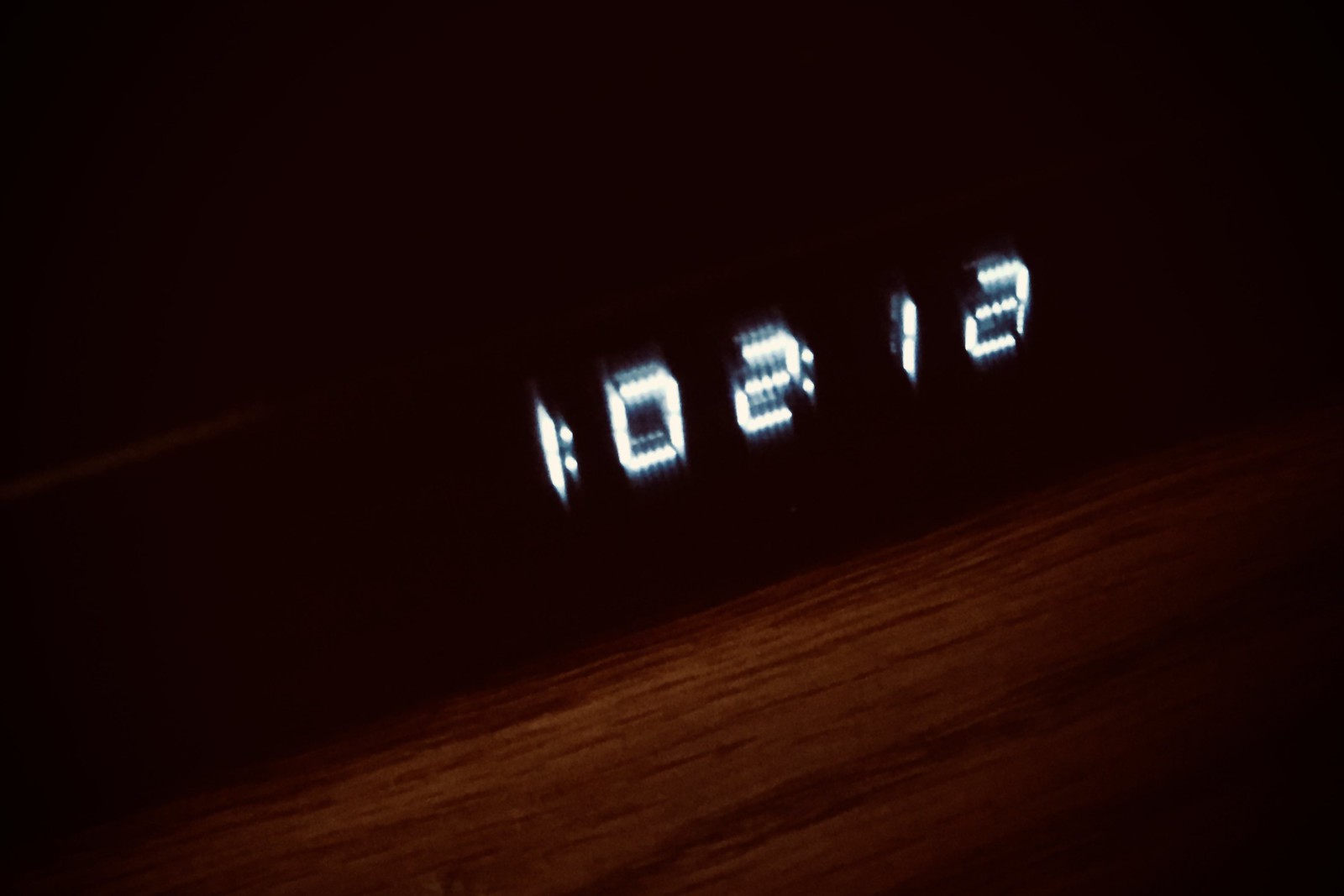The image shows a wooden background that occupies the bottom half, extending diagonally from the left-hand corner to about halfway up the right-hand side. The wood in this section features a noticeable grain pattern. Above this, there is a darker, almost solid brown section that contrasts with the wood grain below. Diagonally across this darker section, there are numerical markings that read "1:02," followed by a gap, and then continue with the number "12." The purpose or meaning of the scene remains unclear.